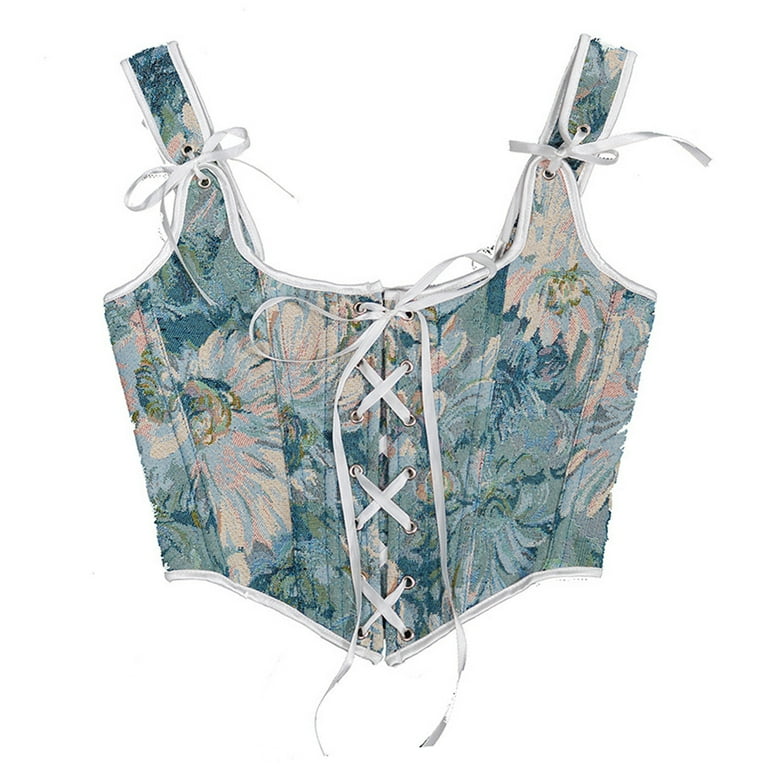This image depicts a corset-style top featuring a vibrant, multicolored floral pattern with abstract flower shapes in light blue, pink, and other floral hues. The garment has thick straps that are tied at the shoulders with delicate white ribbons, forming neat bows. The front is intricately designed with crisscross laces, secured by three sets of white shoelace-like ties that culminate in a bow at the top. Edged with a fine white trim around the top, bottom, and straps, the corset is not full-length, coming down to about half the torso and ending in an angular shape. The fabric appears robust and sturdy, suggesting it is made to provide a certain level of support.